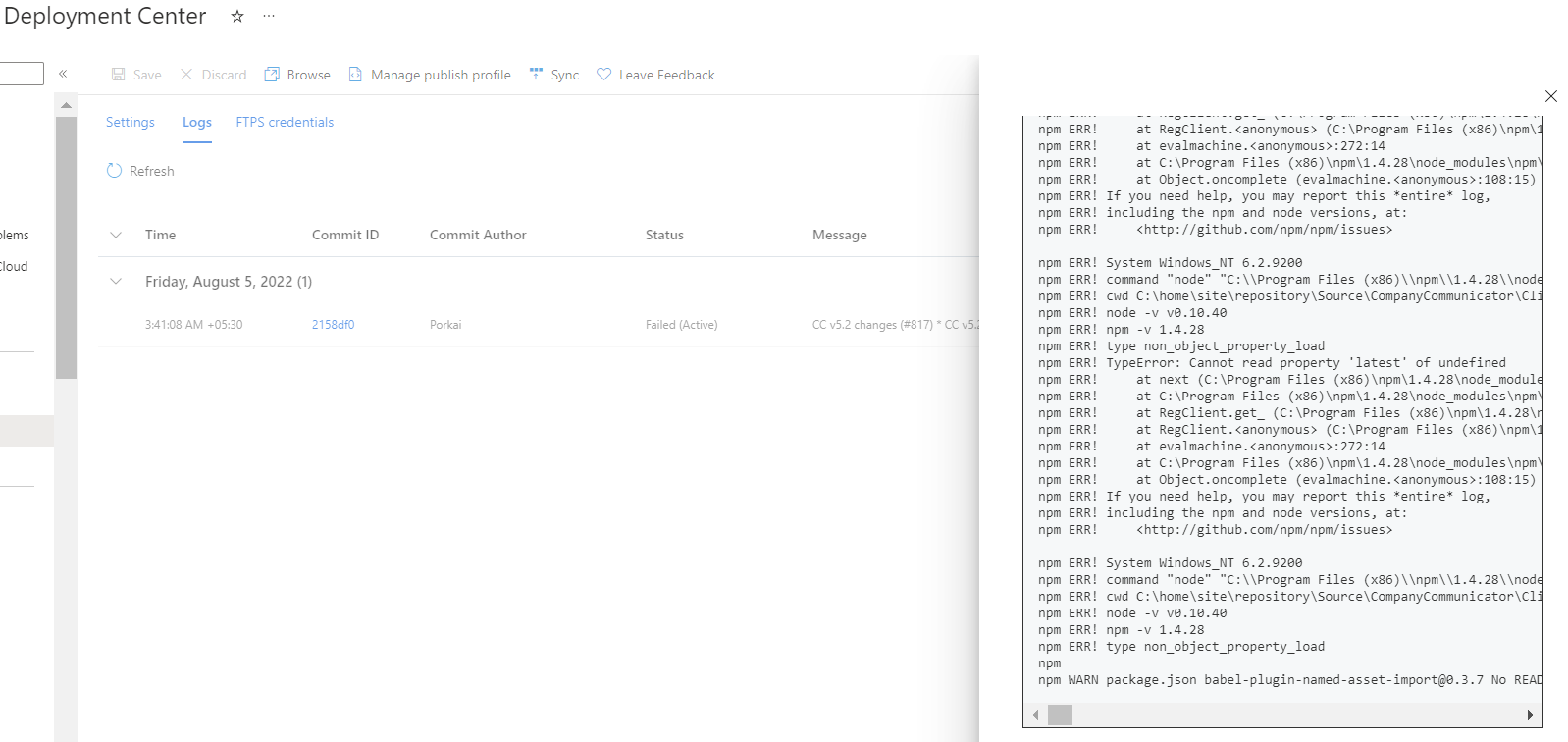The image depicts a form titled "Deployment Center" at the top, highlighted in black font against a white background. Below the heading, there is a star symbol followed by three small dots. The first line beneath "Deployment Center" contains several icons, though their specific details are unclear. There is also a line with an arrow indicating that the page can be scrolled up or down. Following this, there are blue subheadings in a very light and small font. To the right of the subheadings, there appears to be an information sheet that resembles a newspaper due to its densely packed and very tiny text, further suggesting it contains detailed deployment-related information.